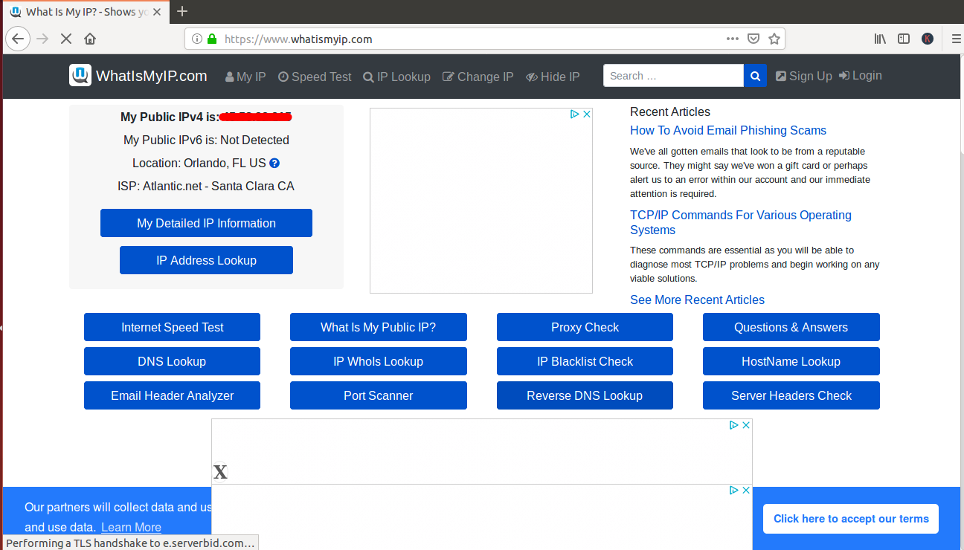The image showcases the homepage of the website "whatismyip.com". At the top of the page, there is a menu bar featuring the site's logo on the far left, followed by the title "whatismyip.com." The menu items listed are "My IP," "Speed Test," "IP Lookup," "Change IP," "Hide IP," a search bar, and options to "Sign Up" and "Log In," each accompanied by a small icon.

The main section of the homepage is populated predominantly with buttons and text, and it lacks visual images. A pop-up at the bottom prompts users to "Click here to accept our terms," with additional advertisement pop-ups also appearing at the bottom of the page.

The buttons on the homepage lead to various tools and features: "My Detailed IP Information," "IP Address Lookup," "Internet Speed Test," "What is My IP," "Proxy Check," "Questions and Answers," "DNS Lookup," "IP Blacklist Check," "Host Name Lookup," "Email Header Analyzer," "Port Scanner," "Reverse DNS Lookup," and "Server Headers Check."

In the top right corner of the page, there's a section titled "Recent Articles," providing users with the latest informational content.